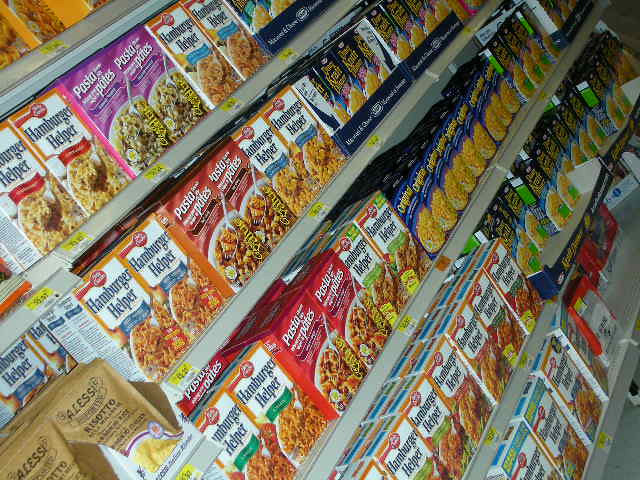The photograph captures a segment of a grocery store aisle, viewed from an oblique angle, emphasizing a section laden with various meal preparation products. On display are multiple shelves, specifically stocked with boxes of Hamburger Helper, diverse pasta varieties, and other meal convenience items. There are six fully loaded shelves, each brimming with an assortment of boxed goods.

In the immediate foreground, prominently attached to the shelves housing the Hamburger Helper boxes, is a cardboard container holding flexible, sealed pouches of Elisi Risotto, adding a touch of variety to the product range.

As the eye moves from the foreground to the background, the selection of Hamburger Helper slowly transitions to several shelves stocked with iconic blue boxes of Kraft Macaroni & Cheese Dinners, completing the rich tableau of meal essentials.